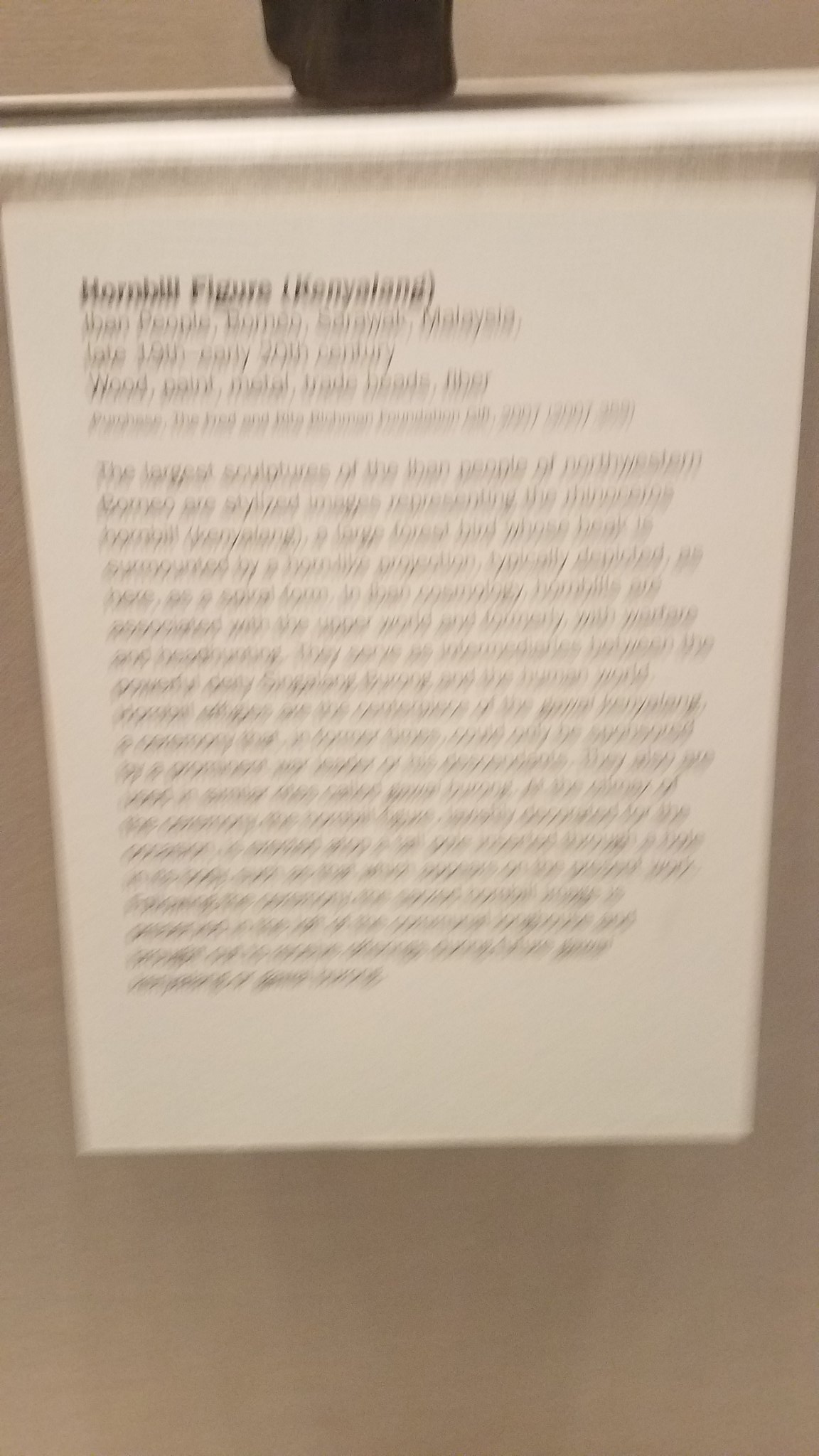This sepia-toned photograph features a slightly grayish background with an unfocused label prominently displayed in the center. The label stands out due to its lighter color compared to the background. While the text is illegible, its structure is discernible. At the top of the label, a headline consisting of three words is visible but remains unreadable due to the small print. Below this headline, there are four to five lines of text, followed by a paragraph space and then a more extensive block of solid text. At the very top of the label, there appears to be a dark-colored element resembling a knob. The overall image exudes a vintage aesthetic, enhanced by the sepia tone and the blurred details.